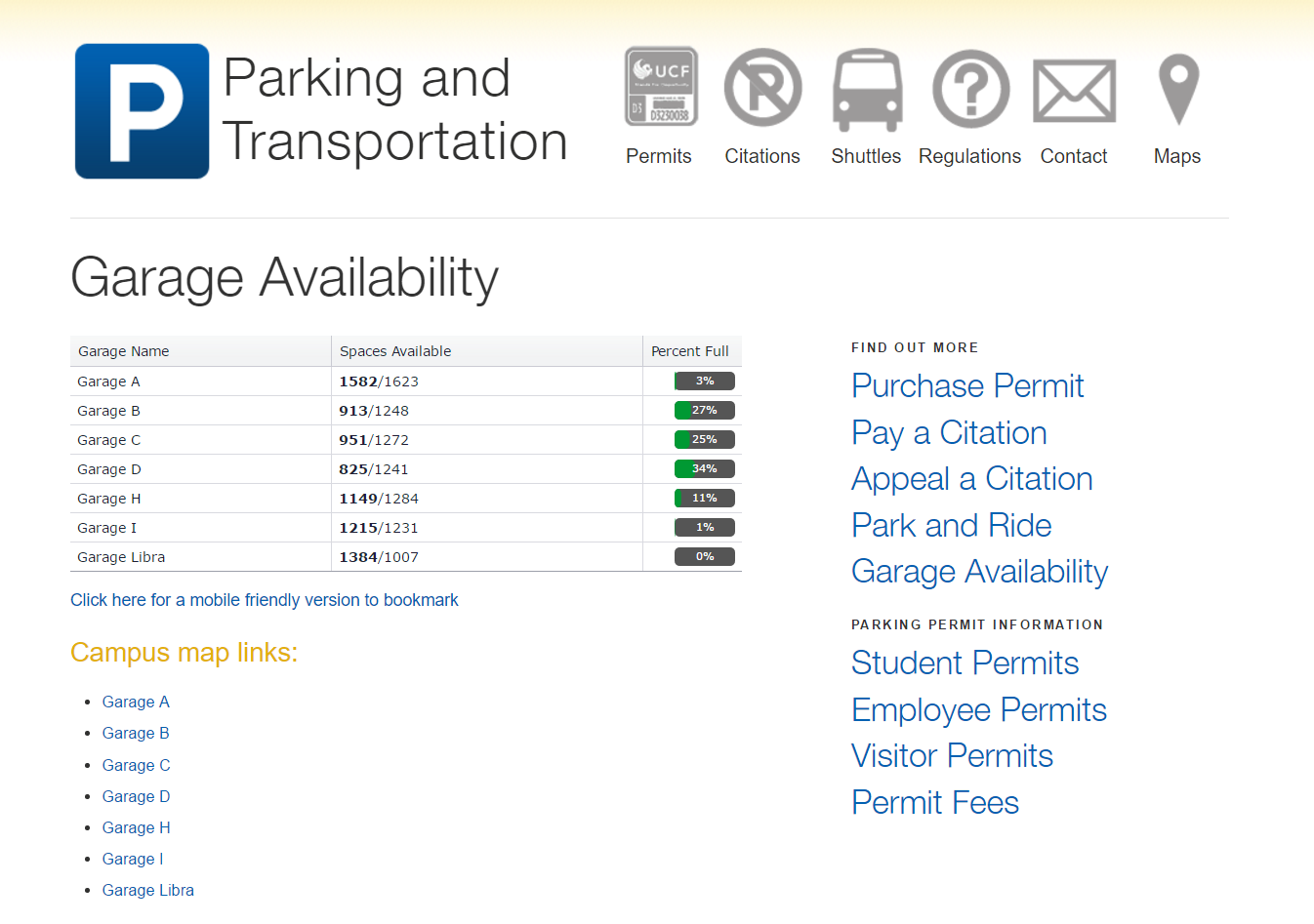The image showcases a detailed webpage dedicated to parking and transportation information for the University of Central Florida (UCF). The page prominently features a blue square with a white 'P', indicating instructions for parking. The heading and various sections are highlighted with orange text, and include links to critical areas such as a campus map and garage availability. The garages listed are A, B, C, D, H, I, and Libra, each providing detailed occupancy percentages.

There are icons and links for tasks and information including purchasing permits, paying citations, appealing citations, and viewing garage space availability. Various user options are categorized under student permits, employee permits, visitor permits, and permit fees. A significant portion of the page also allows users to access maps, contact information, shuttle regulations, and more.

The background is predominantly white with gray and black accents at the top, creating a clean and straightforward interface. Users are offered a mobile-friendly version and can easily bookmark the page for future reference. Overall, the page presents a structured and user-friendly layout for managing parking and transportation needs at UCF.